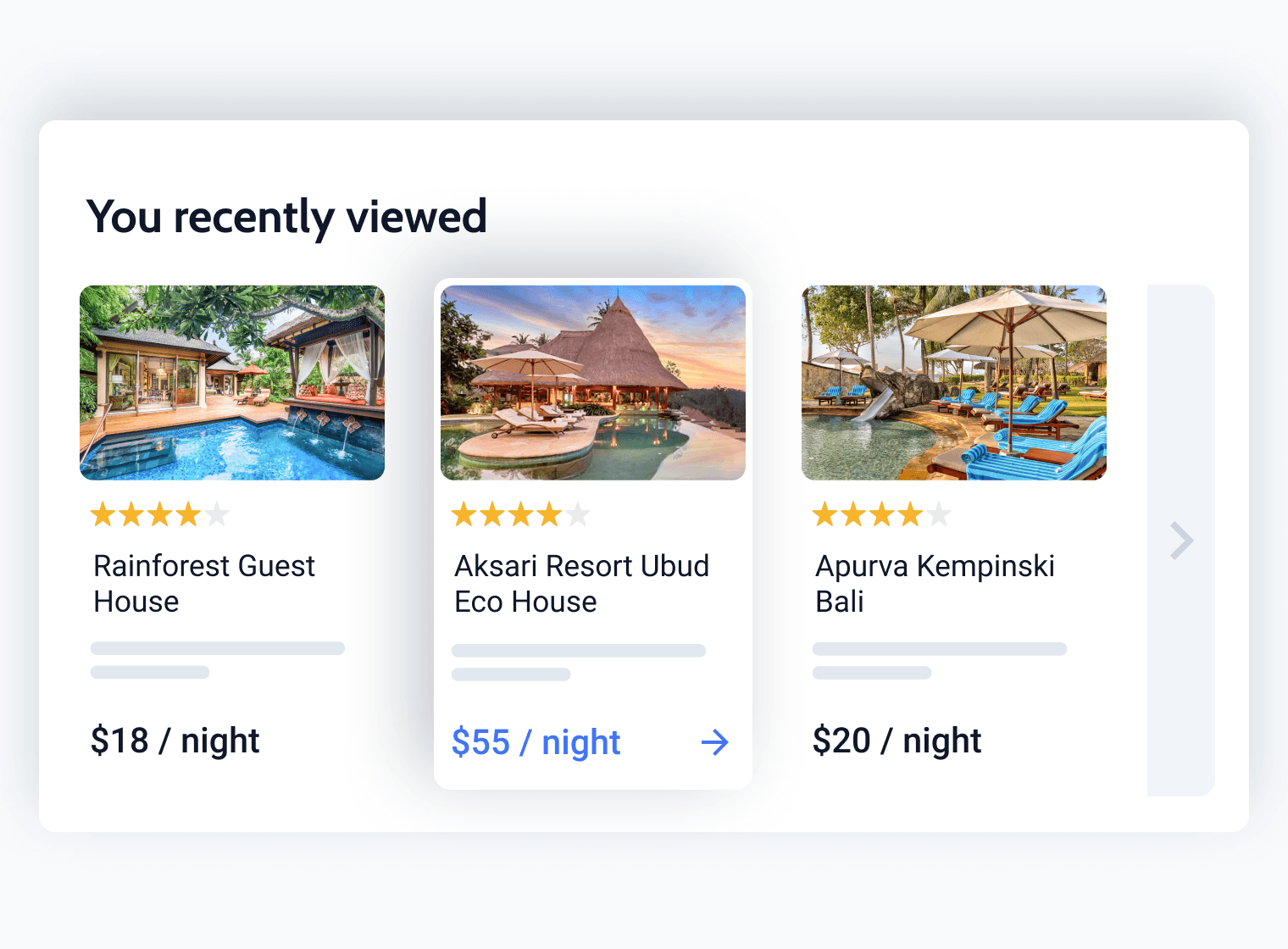The image presented is a screenshot from a travel or hotel booking website displaying recently viewed properties. The overall background is gray, featuring a lighter gray or white pop-up bubble. In the top left corner of the pop-up, black text reads "You recently viewed." Below this header, the pop-up displays three recently viewed hotel properties.

1. On the left, there is an image of a lush pool area surrounded by abundant greenery and a few cabanas. This property, named "Rainforest Guest House," has a rating of four out of five stars and is priced at $18 per night.

2. The middle section highlights "Aksari Resort Ubud Eco House," indicated as being currently selected. The image shows a tranquil pool with pool chairs under umbrellas and a cabana with a grass roof. This property also boasts a four-star rating and is priced at $55 per night.

3. On the right, the image displays a pool area featuring several beach chairs equipped with towels and umbrellas, along with a visible water slide. This property, "Apoorva Kempinski Bali," is similarly rated four out of five stars and is listed at $20 per night.

Each listing is clearly presented with visual appeal and pertinent details to aid in the user's selection process.